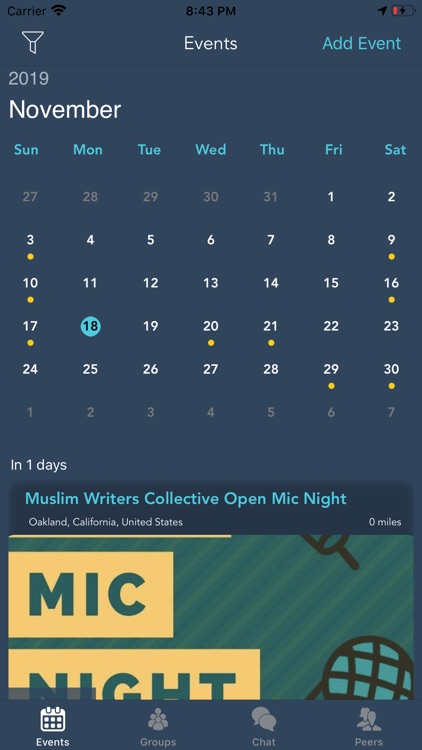This is a screenshot from a cell phone displaying a calendar app. The header is a dark gray with the year "2019" prominently featured beneath a small funnel icon. The words "Events" are written in white across the top, and to the right, there’s a blue "Add Event" button. Below this header, the calendar is set to November 2019, with "November" labeled in white. The calendar grid displays the days of the week abbreviated as Sun, Mon, Tue, Wed, Thu, Fri, and Sat, with days of the week highlighted in blue. The month starts on a Friday, and the dates are marked in white, except for the dates belonging to October and December, which are in gray. Additionally, some dates feature yellow dots signifying events, such as "Mike Knight, Muslim Writers Collective Open Mike Knight."